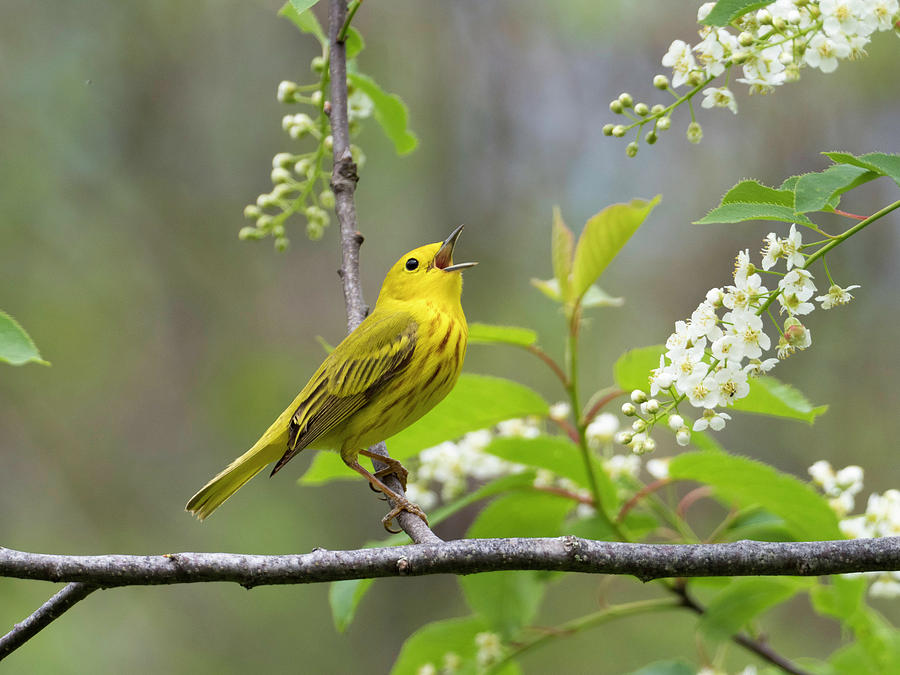This captivating landscape-oriented photograph captures a vivid scene of a yellow bird, specifically a Yellow Warbler, perched on a tree branch. The bird, predominantly bright yellow with greenish-yellow wings tipped with subtle streaks of brown, is facing to the right with its beak open as if mid-song, revealing its black eyes and characteristic warbler markings. The focal tree branch stretches horizontally across the lower part of the image, with the smaller twig intersecting upward where the bird is perched. Surrounding the Yellow Warbler are delicate clusters of small, white flowers with yellow centers, accompanied by green leaves, creating a picturesque floral backdrop. The background seamlessly transitions into an out-of-focus grayish-green, emphasizing the vibrant colors of the bird and flowers. The photograph embodies representational realism, capturing the intricate details and natural beauty of the bird and its environment in a serene outdoor setting.